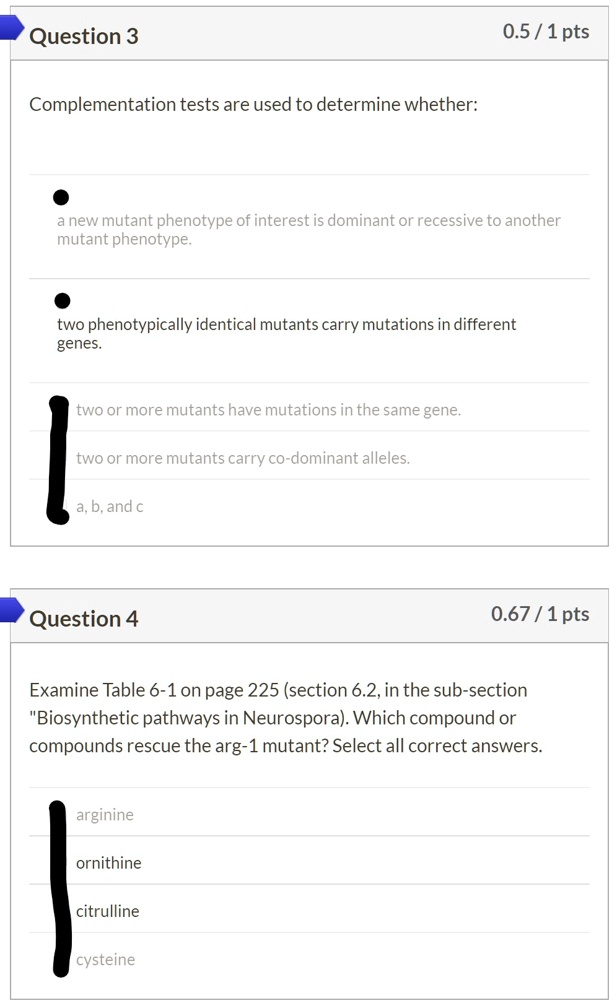This is a detailed description of a screenshot taken from a mobile testing platform. The screenshot displays two questions, labeled as Question 3 and Question 4, each with corresponding points indicated next to them, though it is uncertain whether these points reflect the value of correct answers or the points awarded to the test taker for their responses. 

At the top of the screenshot, a statement reads: "Contemplation tests are used to determine whether-". The answers provided for this stem include:

1. A new mutant phenotype of interest is dominant or recessive to another mutant phenotype.
2. Two phenotypically identical mutants carry mutations in different genes.
3. Two or more mutants have mutations in the same gene.
4. Two or more mutants carry co-dominant alleles A, B, and C.

Question 4 details a specific instruction: "Examination table 6-1 on page 225 section 6-2 in the subsection biosynthetic pathways and neurospora. Which compound or compounds rescue the ARG1 mutant? Select all correct answers." The answer choices for this question are:

- Arginine
- Ornithine
- Citrulline
- Cytine

Notably, all the answer selections are manually blacked out, likely using a tool such as Microsoft Paint or a similar touch-screen application, which was possibly done by the person who took the screenshot to obscure their selected answers.